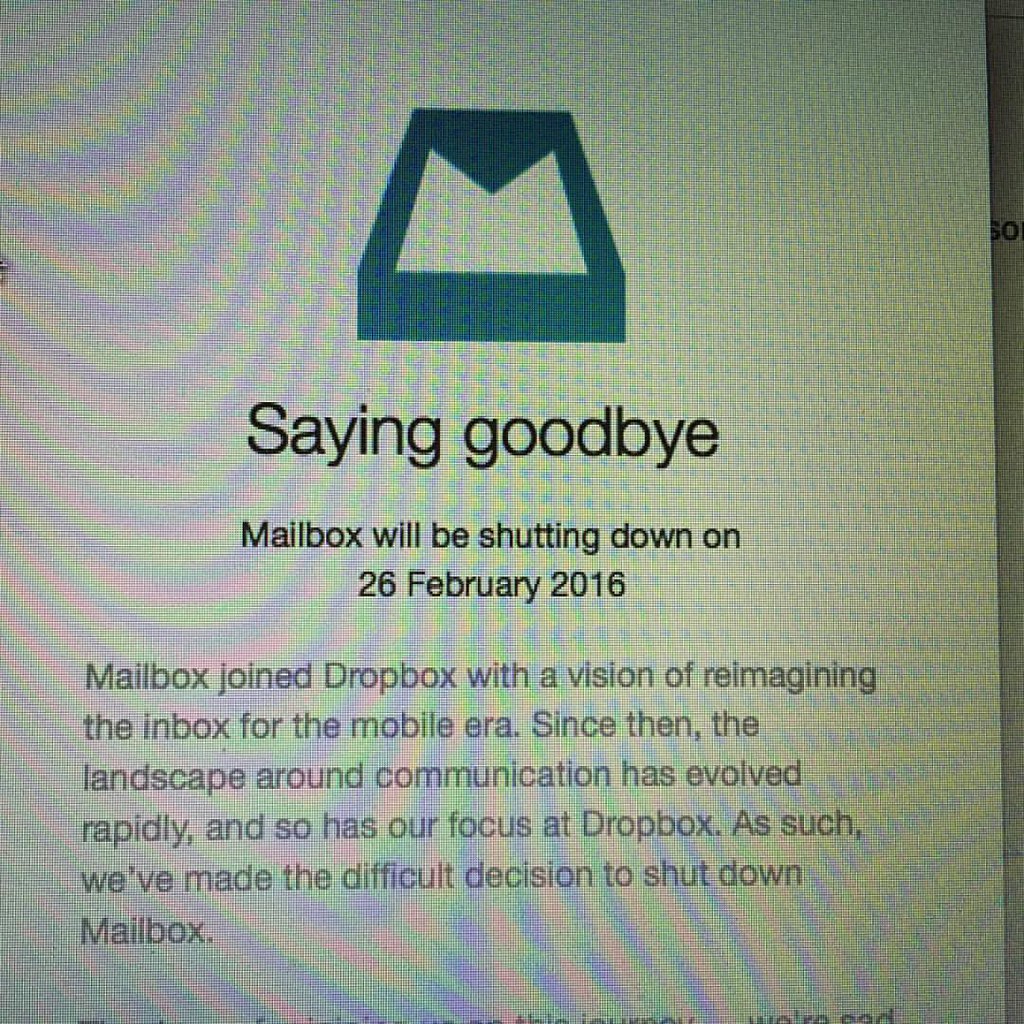The image is a photograph of a computer screen, exhibiting visible digitized glare and a rainbow pattern across the top left corner, typical of a camera-captured screen image. The central focus of the image is an online alert from Mailbox, an application tied to Dropbox. The alert reads: "Saying Goodbye. Mailbox will be shutting down on 26 February 2016." Beneath this, in gray text, it explains, "Mailbox joined Dropbox with a vision of reimagining the inbox for the mobile era. Since then, the landscape around communication has evolved rapidly, and so has our focus at Dropbox. As such, we've made the difficult decision to shut down Mailbox." A portion of additional text is visible at the very bottom but is mostly cut off, hinting at an expression of sadness regarding the shutdown. A small icon representing Mailbox can be seen at the top of the screen.